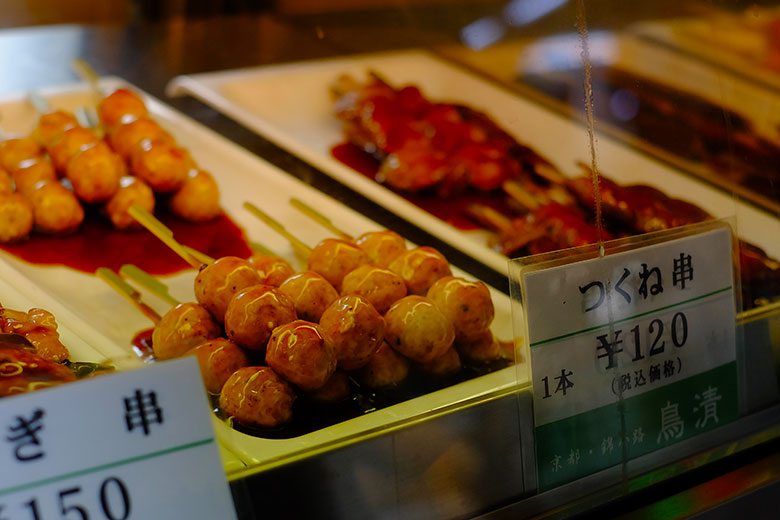The image shows a close-up view of several food items displayed behind a glass counter, likely in a Japanese supermarket or food section. The food items are arranged in white trays. On the left side, there are skewers with three chicken meatballs each, covered in a savory sauce. To the right, there are skewers with what appears to be teriyaki or yakitori, possibly chicken or pork. The tray at the front shows a price tag of 150 Japanese yen for the meatballs, while the skewers on the right display a price tag of 120 yen. The labels have white tops and green bottoms with black Japanese text. The food looks appetizing with a glossy layer of oil or sauce, and the overall setting suggests a clean, organized display typical of a Japanese food market.